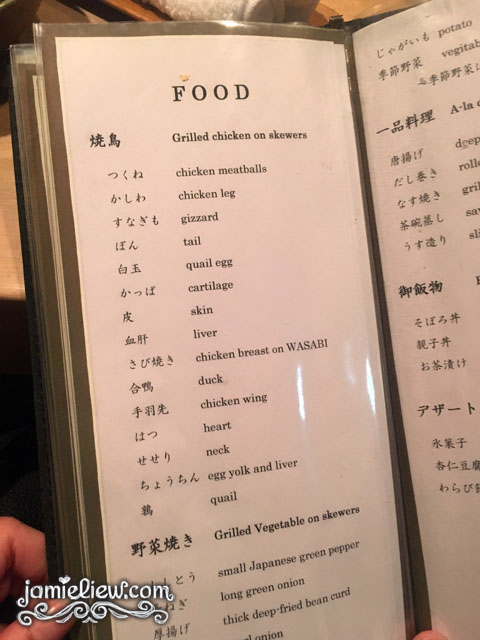This detailed image showcases a page from a Japanese restaurant's menu, with the website "jamielou.com" elegantly inscribed at the bottom. Below the site address, intricate designs grace the space, adding a touch of artfulness. Notably, the letter "i" in "Jamie" features a charming heart symbol as the dot. This particular menu page is dedicated to various grilled dishes, prominently labeled "Food" at the top. 

The menu lists an array of grilled chicken options, including skewers of chicken meatballs, leg, gizzard, tail, wing, heart, neck, skin, liver, breast with wasabi, and cartilage. It also offers more exotic choices like quail eggs, duck, egg yolk, and liver. For those preferring something other than meat, there is an assortment of grilled vegetables, featuring small Japanese green peppers, long green onions, and thinly sliced deep-fried bean curd. 

The menu is bilingual, presenting the Japanese names of the dishes on one side with their English translations clearly provided on the other, ensuring clarity and accessibility for all patrons.